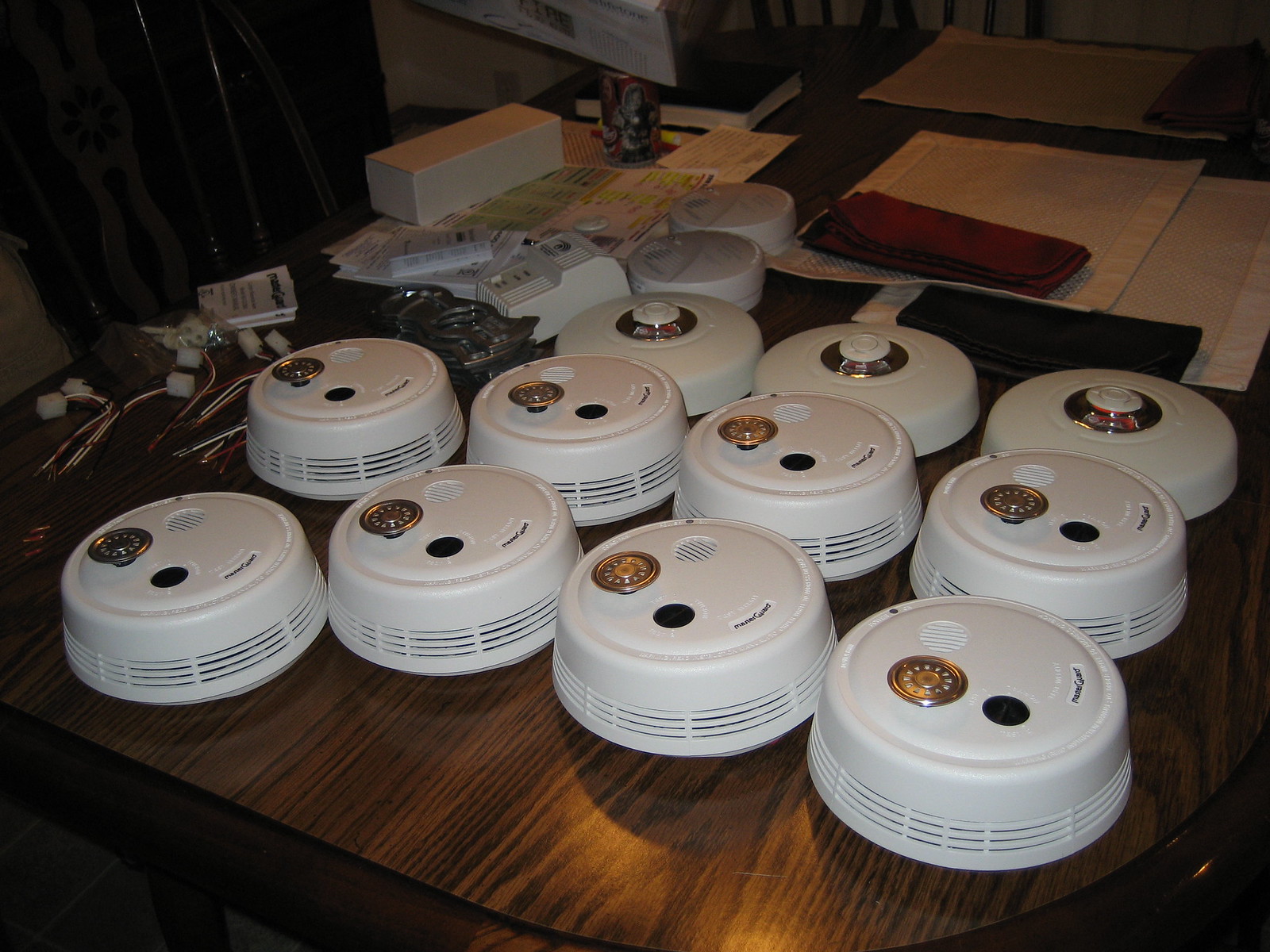This is a detailed photograph of multiple smoke detectors and possibly carbon monoxide detectors displayed on an oval, brown wooden table with curved edges. There are eight prominent large detectors at the forefront, each featuring a gold metal circle, a smaller black button, and apparent vents along the bottom. Positioned in three neat rows, these devices are roughly three inches tall and appear uniform with white plastic casings. Behind these main detectors are three additional white, round devices with a white plastic cap on top, possibly a different type of detector. Scattered around the table are two smaller white smoke detectors without knobs or buttons. The background of the image shows an assortment of items, including wires, several instruction sheets, white fabric placemats, folded black or maroon-colored napkins, a red eyeglass case, and some strewn papers, adding a cluttered element to the scene.